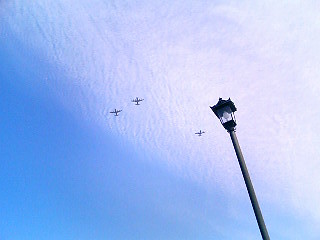This detailed photograph captures a captivating scene from the ground, looking up at a clear blue sky with scattered cirrus clouds. Three small airplanes are visible in the middle of the frame, flying in an informal but close formation, suggesting they might be part of an air show or a military exercise. The planes appear quite distant and lack detailed features due to their altitude. The left portion of the sky is predominantly blue, while the right portion transitions to white with more clouds. On the right side of the photo, a tall street lamp, unlit due to the daytime setting, rises diagonally toward the left, adding urban context to the aerial display.